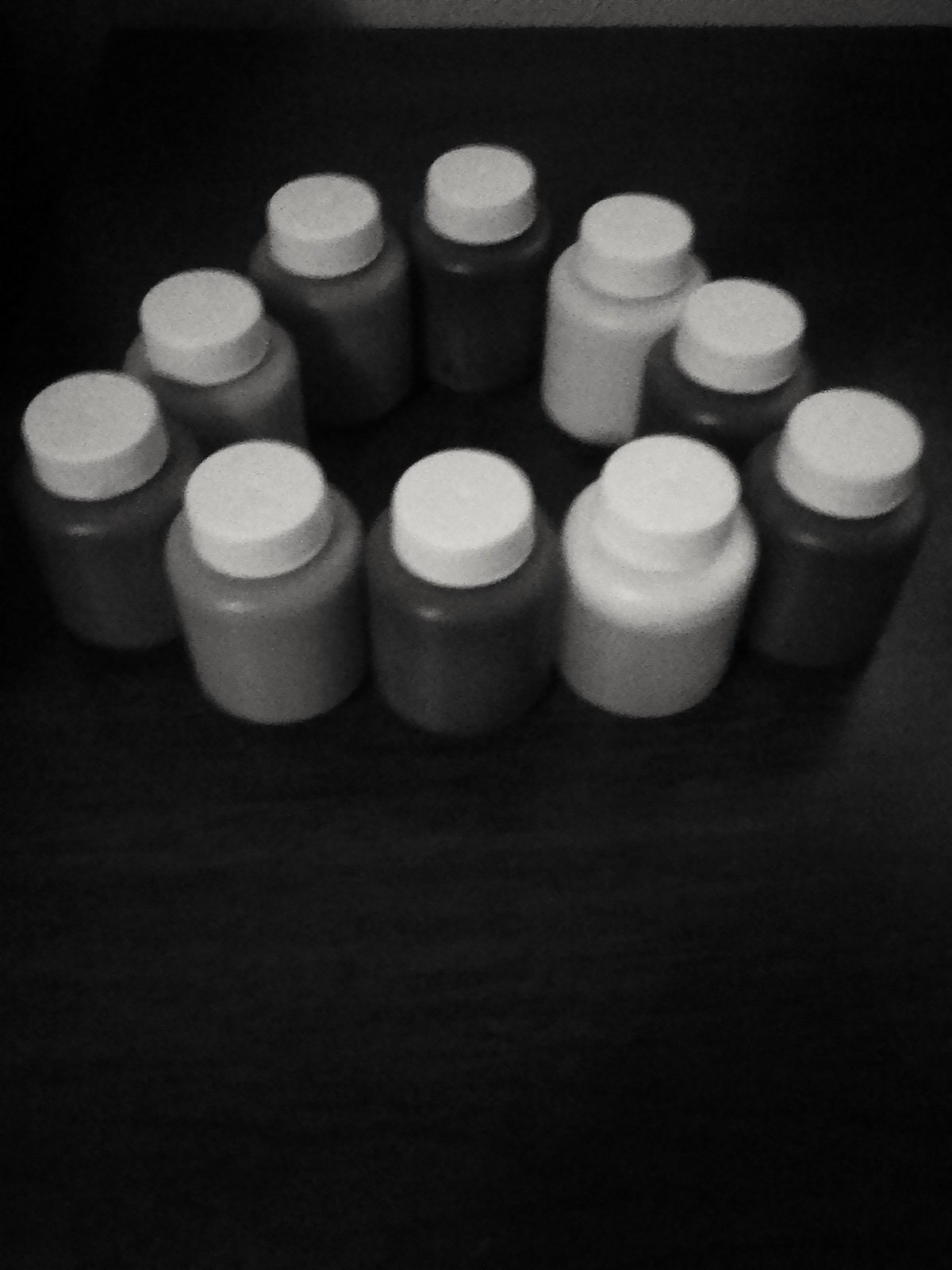This is a detailed black-and-white photograph depicting a collection of artist paint bottles, possibly acrylic, neatly arranged on a table. The background, made of fabric, transitions from a darker black at the top to a lighter shade towards the bottom, creating a subtle gradient. The bottles, ten in total, are small, round, and made of plastic, each topped with a short, squat white cap. The paint bottles are arranged in a geometric shape: a semicircle at the top that complements a straight line of bottles at the bottom, forming a triangular configuration. Although the image is monochromatic, the bottles themselves range in shade from light to dark, with visible variations in grey scale. The distinct details of each bottle – alternating shades of black, white, and grey – provide a focal point against the textured, rippled background fabric that peeks through the arrangement.